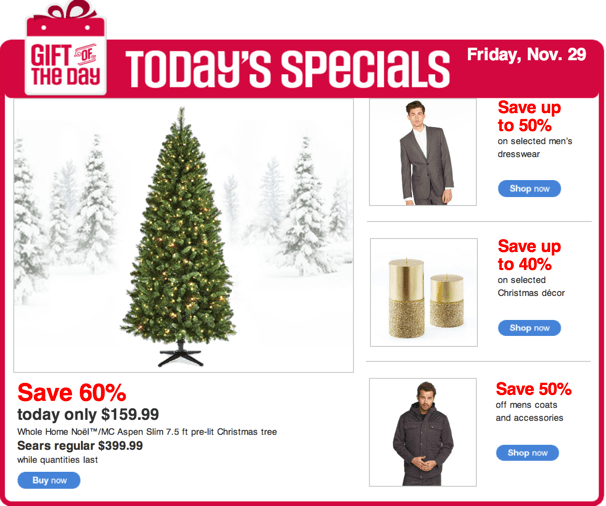Discover incredible holiday savings in this vibrant online advertisement. At the top, a festive red outline surrounds a box featuring a Christmas gift box icon with a bow, titled "Red Gift of the Day." In white text, it announces "Today's Specials Friday, Nov 29."

The central portion of the ad showcases a slightly olive-green artificial Christmas tree adorned with golden-clear lights and set against a background of snowy trees. Highlighted in bold red, the text reads "Save 60%," followed by black text stating, "Today only $159.99." The detailed description continues, "Whole Home Noel Mc Aspen Slim 7.5 feet Pre-Lit Christmas Tree, Sears regular $399.99, while quantities last." A blue and white "Buy Now" button is prominently displayed below.

On the adjacent side, the ad features various images and offers, starting at the top with a dark-haired man in a white shirt and gray suit from Paul Taylor. Below him, a red and black text advertises "Save up to 50% on selected Men's Dress Wear" accompanied by a blue and white "Shop Now" button.

The next image showcases elegant gold candles, with a solid gold top and a sparkly bottom part. The banner highlights "Save up to 40% on selected Christmas decor" along with a blue and white "Shop Now" button.

The final image depicts a male model with brown hair and facial hair, dressed in a dark gray shirt and pants. The caption reads "Save 50% off Men's Coats and Accessories."

Immerse yourself in these exceptional deals and make the most of your holiday shopping!